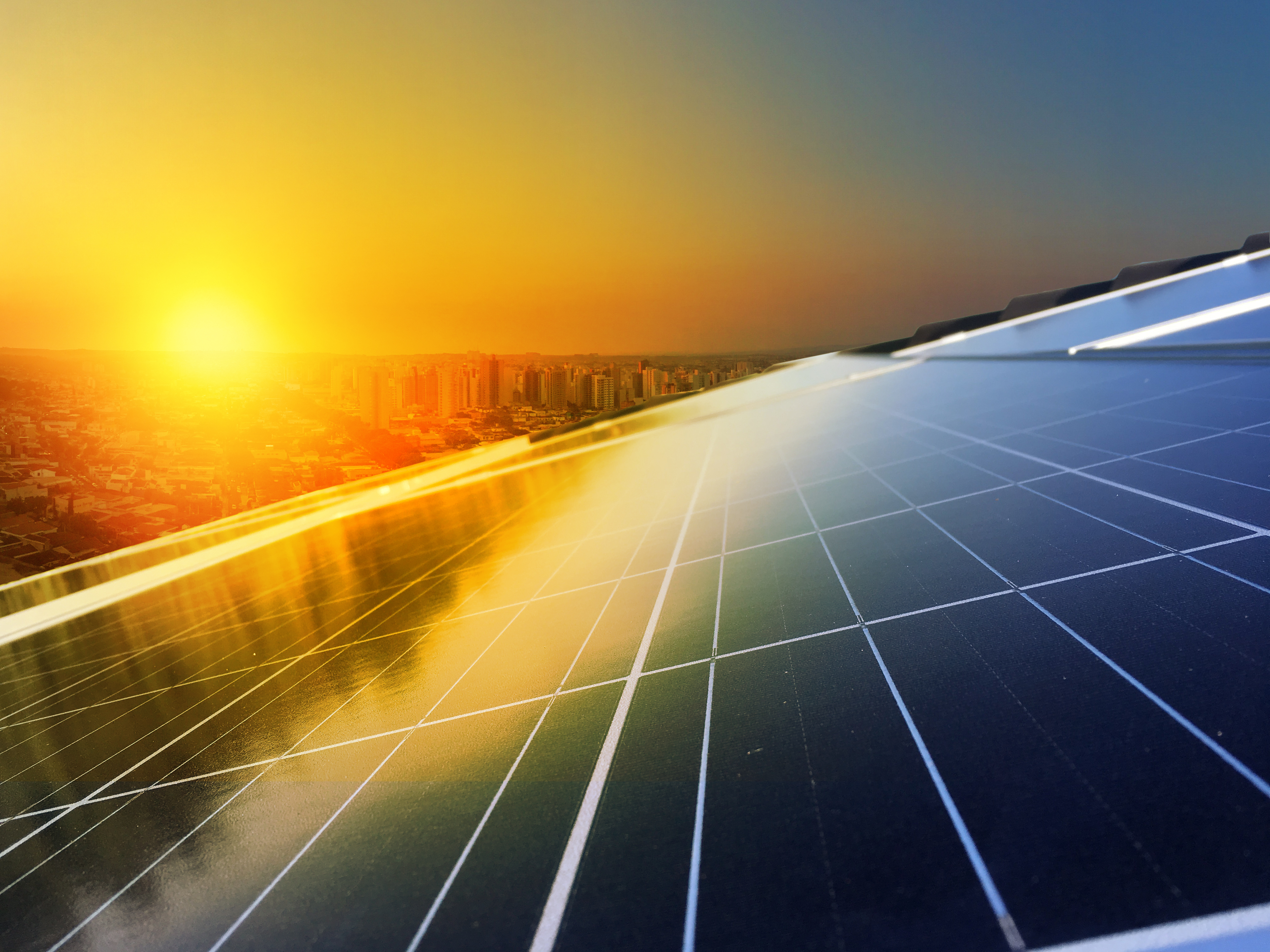The photograph depicts an expansive rooftop adorned with a series of large, glossy solar panels. Taken at either dusk or dawn, the image features the sun half-visible on the horizon, casting a radiant glow that bathes the entire scene in warm hues. The panels predominantly appear black with white grid lines, though the sunlight gives them a yellowish sheen, reflecting the vibrant sky above. To the left, the sky transitions through a gradient of colors from deep blue to lighter blue, and ultimately to hues of yellow, orange, and gold as it meets the horizon. In the far background, high-rise buildings of a sprawling city are visible, colored orange from the sun's early or late rays. The left side of the solar panels even mirrors parts of this cityscape, adding depth to the image. Only a few panels are visible up close, suggesting a slanted rooftop that houses several more. The sky is predominantly clear, enhancing the brilliance of the scene. Major colors in the photograph include rich shades of blue, orange, yellow, and gold, with highlights of white and black.